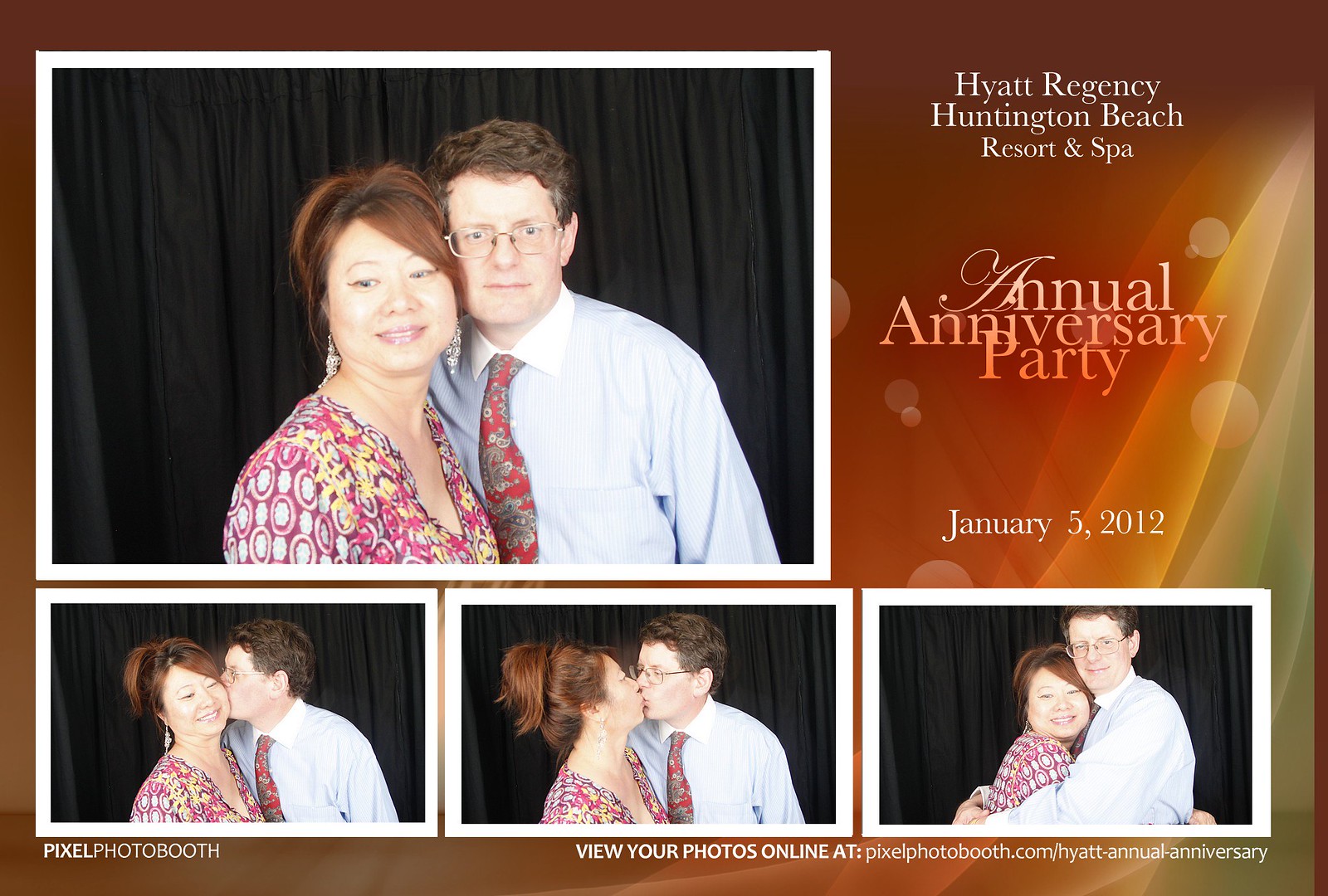The image depicts an invitation or flyer for the "Hyatt Regency Huntington Beach Resort and Spa Annual Anniversary Party" held on January 5, 2012. In the top right corner, this event information is clearly displayed. On the left side of the flyer, the largest photo shows a couple: an Asian woman with medium-length brown hair dressed in a pink, yellow, and white blouse paired with long chandelier earrings, and a white man with dark hair, eyeglasses, and a white button-down collared shirt with a red and green tie. They stand in front of a long black curtain. Below this main photo, there are three smaller images of the same couple engaging in affectionate poses, including hugging and kissing.